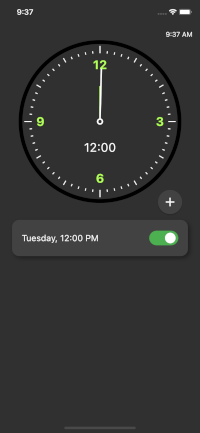The image features a sleek black background. At the very top, it displays "937" followed by "937 a.m." to its right. Dominating the center of the image is a clock with striking yellow-green numbers denoting the 12, 3, 6, and 9 positions, while the other hour markings are represented by white lines. Both white hands of the clock are aligned at the 12, indicating that it is exactly 12 o'clock. Beneath the clock face, there is a small white circle with a plus sign inside it.

Further down, a prominent black button displays "Tuesday 12 o'clock p.m." Inset within this button is a green button marked by a white circle. The top part of the image also includes icons for battery life and internet connectivity next to the time display, ensuring the viewer is aware that it is Tuesday and 12 o'clock p.m. The small green slide button beside the text adds an interactive element to the composition.